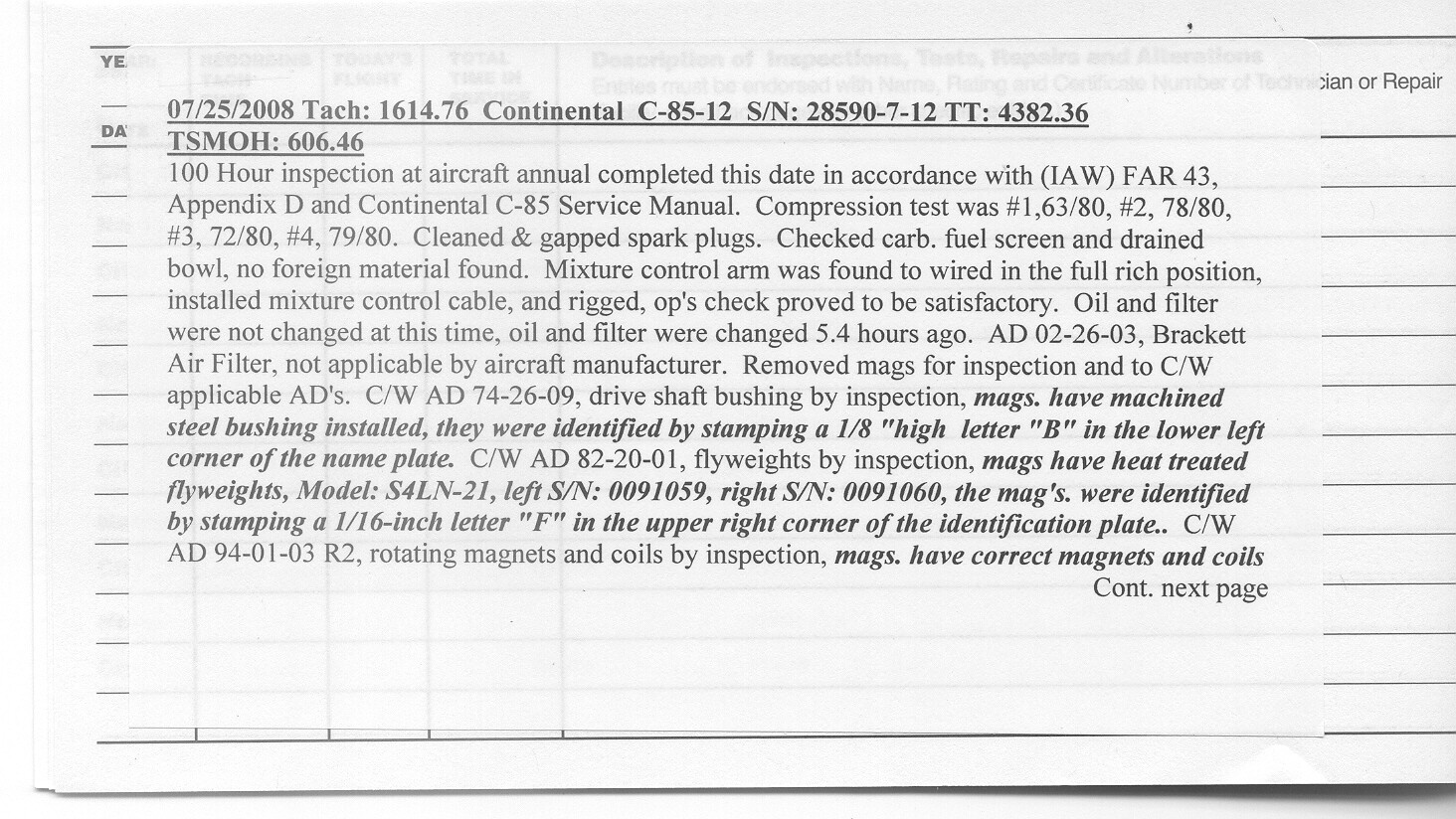This image depicts a white piece of paper featuring black lines with a white square sticker affixed on top. The sticker, printed with small, black text, documents detailed maintenance information for a Continental C-85-12 aircraft engine. Specifically, it reads: "0725-2008 TACH 1614.76 Continental C-85-12S/N 28590-7-12 TT 4382.36 TSMOH 606.46." The sticker describes the completion of a 100-hour inspection and annual maintenance as per IAW FAR 43 Appendix D and the Continental C-85 service manual. A compression test revealed the following readings: #1 63/80, #2 78/83, #3 72/80, and #4 79/80. Maintenance tasks included cleaning and gapping spark plugs, checking the carb fuel screen and drain bowl (with no foreign material found), and addressing the mixture control arm, which was wired in the full-rich position. A new mixture control cable was installed and rigged, with operational checks proving satisfactory. The oil and filter were not changed during this inspection, as they were replaced 5.4 hours prior. Additionally, AD 02-26-03 concerning the air filter was deemed not applicable by the aircraft manufacturer. The magnetos were inspected per several ADs: AD 74-26-09 (drive shaft bushing, identified by a 1/8-inch stamped "B" in the lower left of the nameplate), AD 82-20-01 (heat-treated flyweights for model S4LN-21, with S/N 0091059 on the left and S/N 0091060 on the right, identified by a 1/16-inch stamped "F" in the upper right of the identification plate), and AD 94-01-03 R2 (rotating magnets and coils). The document continues onto the next page.